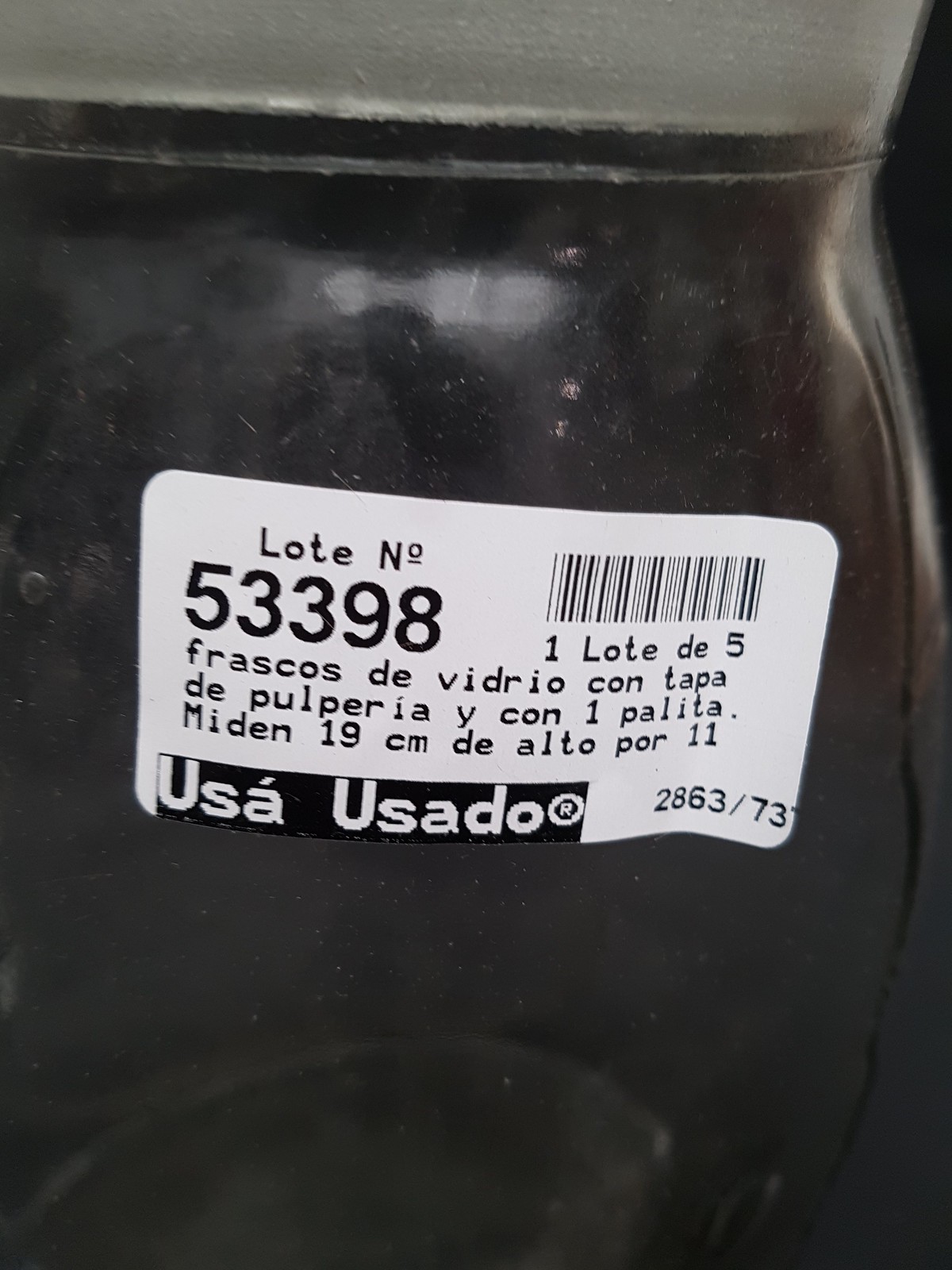The photo features a close-up of a partially visible glass jar adorned with a detailed white label. The prominent elements include a lot number, 53398, and a barcode 53398, one lot D5. Notably, the label is written in Spanish and includes the text: "Frascos de vidrio con tapa de pulperia y con una palita," which translates to "glass jars with pulperia lids and a little shovel." The jar's dimensions are specified as 19 centimeters in height and 11 centimeters in diameter. The label also indicates that the manufacturer is associated with the USA DOE, featuring a registered trademark, "USADO ® 2863/73." The image captures the texture and reflection of the clear glass against a dark background, emphasizing the jar's commercial packaging attributes.